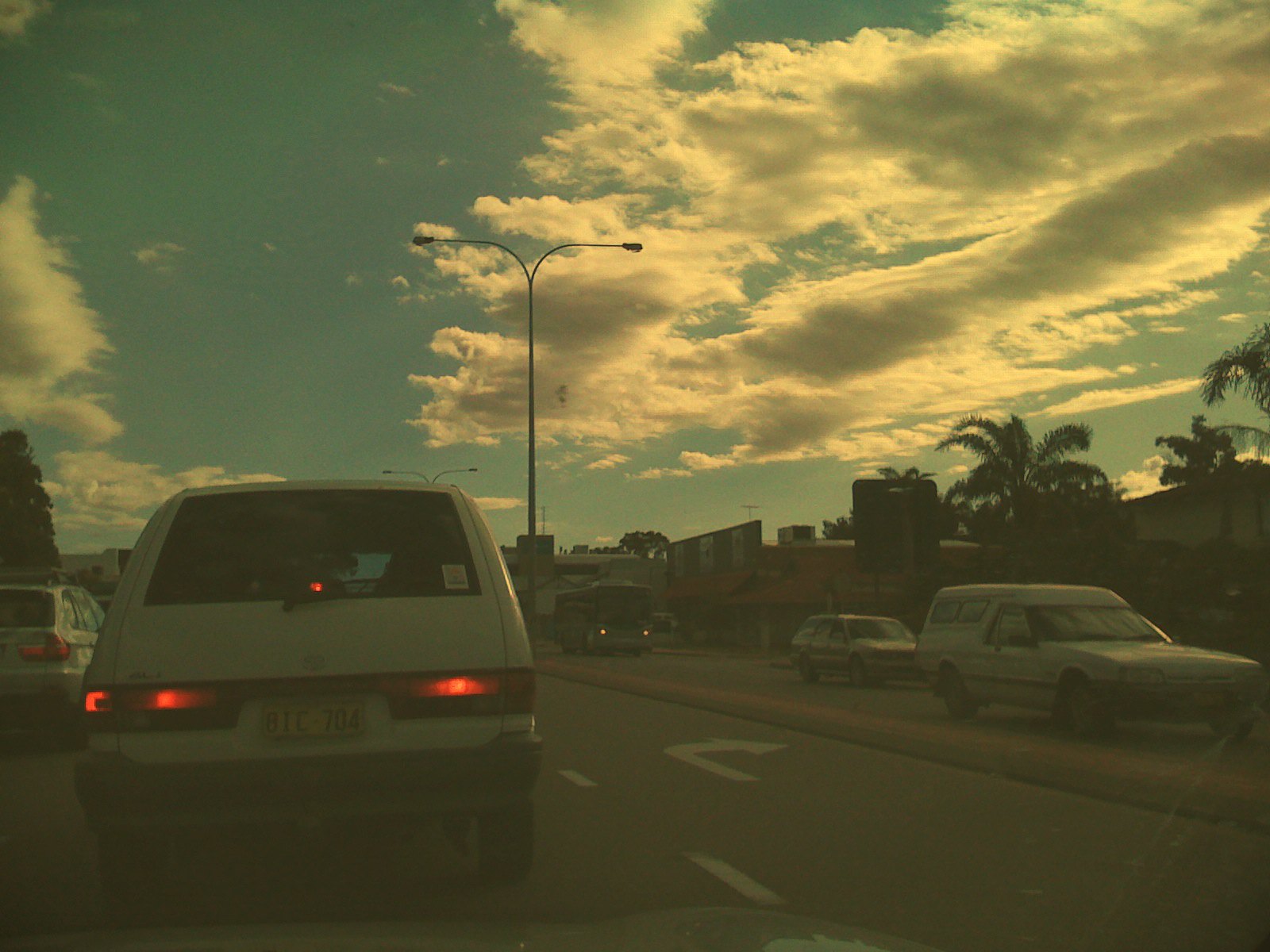The image captures a city street at dusk, imbued with a gentle, dusky filter that gives it an ethereal quality. The photograph is taken from within a car, providing a viewpoint that looks outward and slightly upward. A vast sky, reminiscent of the whimsical skies from "The Simpsons," is painted in varying hues of blue with light and dark clouds intermingling. Dominating the foreground is a large street lamp, casting a subtle glow over the scene. Just ahead is a white car, its brake lights glowing intensely red.

The street's layout is clearly visible, marked by a turn lane and other lane indicators. In the distance, elegant palm trees are faintly discernible, providing a touch of natural beauty against the urban environment. To the left of the composition, a bus is present, adding a dynamic element to the frame. On the right side, the lanes are occupied by two additional cars, their presence adding to the bustling yet serene ambiance of the moment.